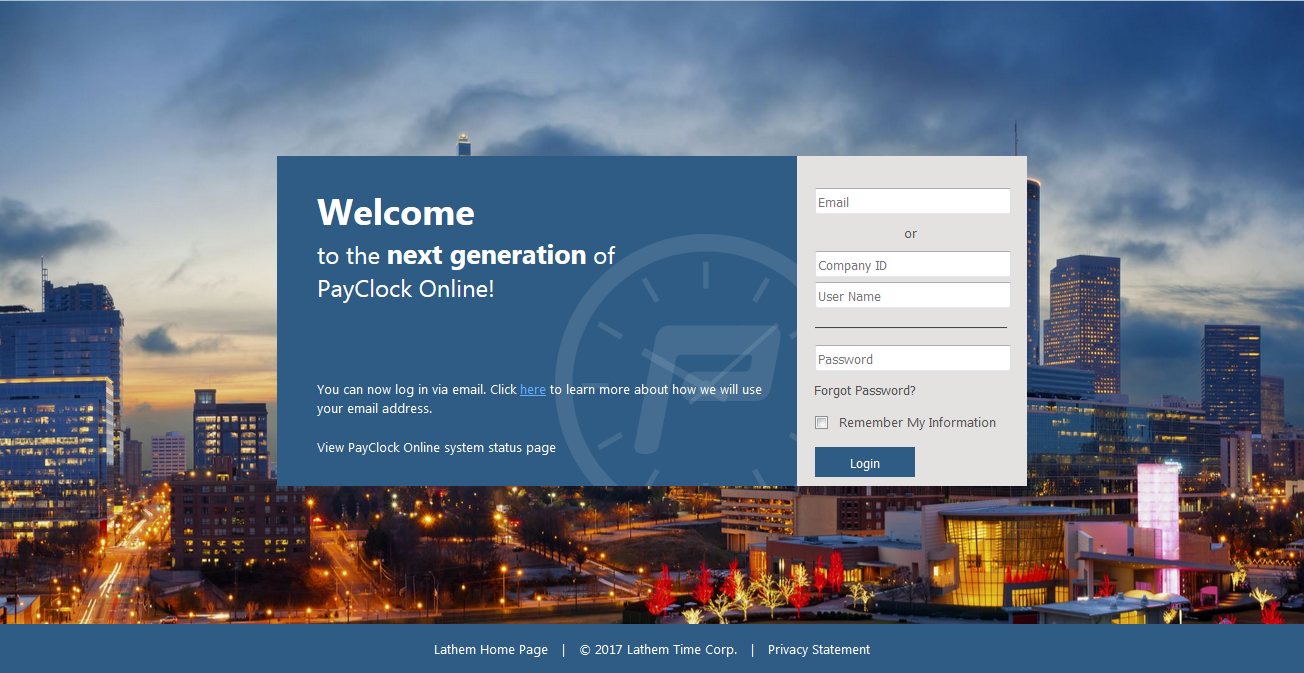The image showcases the homepage for the PayClock Online login system by Lathurn TimeCorp. Dominating the image is a pristine, modern interface inviting users to "Welcome to the Next Generation of PayClock Online." In the center of the screen is a pop-up login form, prompting users to enter their email, company ID or username, and password. The form’s text fields are presented in a bluish hue, complemented by a call-to-action note reading, "You can now log in via email. Click here to learn more."

The backdrop contrasts the modern interface, featuring a vibrant nightscape of a large, bustling city. The illuminated cityscape is dotted with towering office buildings and skyscrapers, with numerous cars weaving through the streets below. Among the skyline, a uniquely pink-lit building stands out, adding a distinctive touch to the urban scenery. The overall backdrop could imply the location of Lathurn TimeCorp’s offices, embodying a sense of modernity and efficiency.

In the upper portion of the image, the logo for Lathurn TimeCorp is visible: a stylized watch dial with a P at its center, featuring hands that circle the letter. This is accompanied by the copyright statement "2017 Lathurn TimeCorp," along with a mention of their privacy statement, solidifying the webpage's identity and credibility.

A subtle part of the background includes greenery with yellow and red trees, suggesting a seasonal transition possibly around fall, contributing to the aesthetic appeal without any overt holiday indications.

Overall, the detailed elements combine to create a user-friendly and visually appealing login interface for the PayClock Online system, reflecting a balance of technological advancement and urban sophistication.